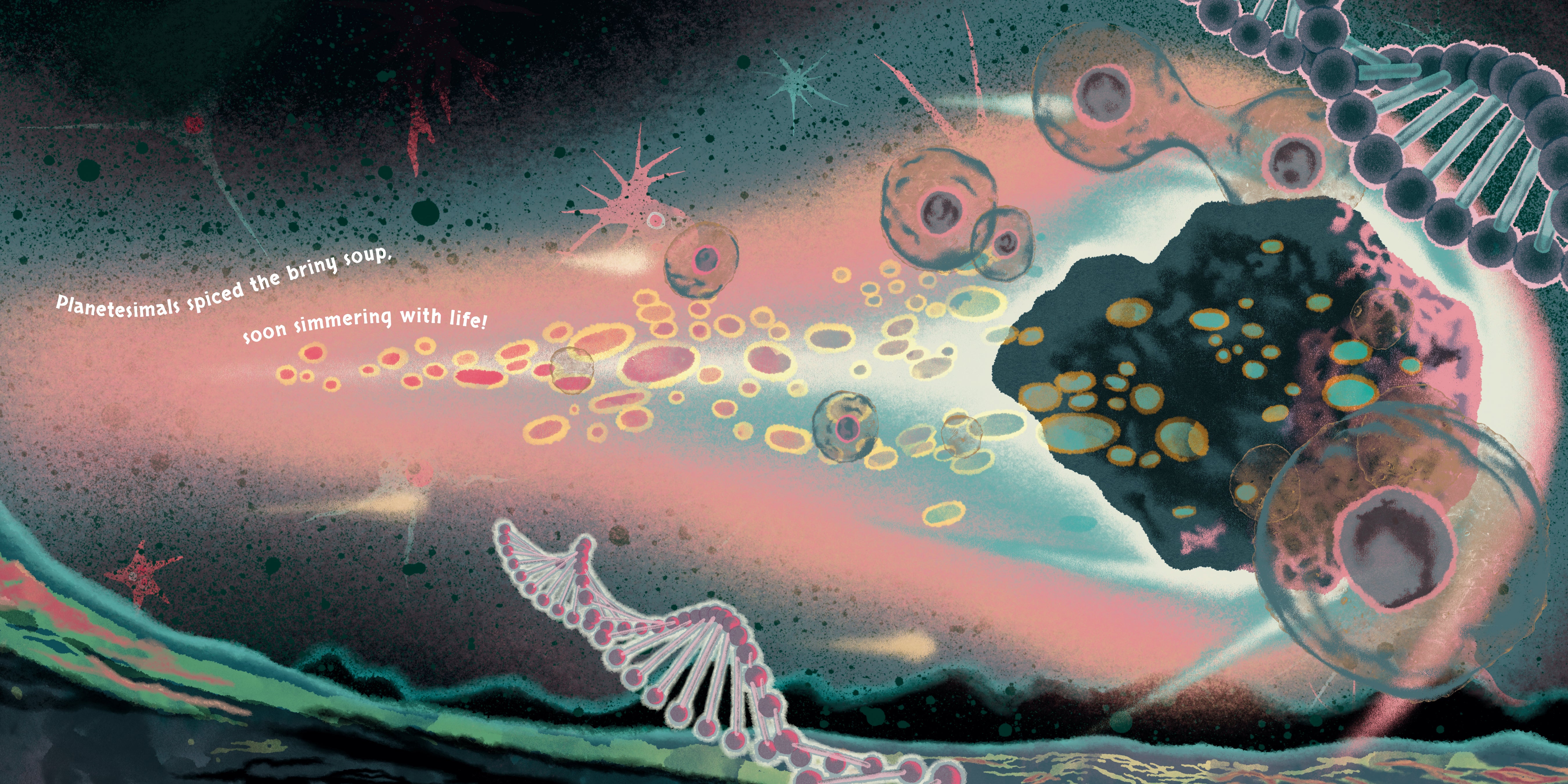The image depicts a detailed, otherworldly scene that appears hand-drawn or painted, resembling something from a scientific textbook. The background is predominantly dark, with a light greenish and dark blue DNA molecule situated in the upper right corner. Streaks of light pink and green colors add contrast throughout the composition. At the bottom of the image, dark blue rocks are adorned with yellow and green ovals and circles. A purple DNA molecule is prominently featured towards the middle bottom, encircled by various shapes and elements that suggest an underwater or extraterrestrial environment. On the left side, pink stars ascend with hints of teal stars trailing upwards. The artwork is imbued with a narrative, as it includes the words "Planet Nesmo spiced the briny soup, soon simmering with life." Among the visual elements, there are also amoeba-like forms with numerous legs and rock formations that hint at biological and geological features. The color palette, featuring shades of pink, teal, peach, and yellow, enhances the scientific yet fantastical nature of this imagined landscape.